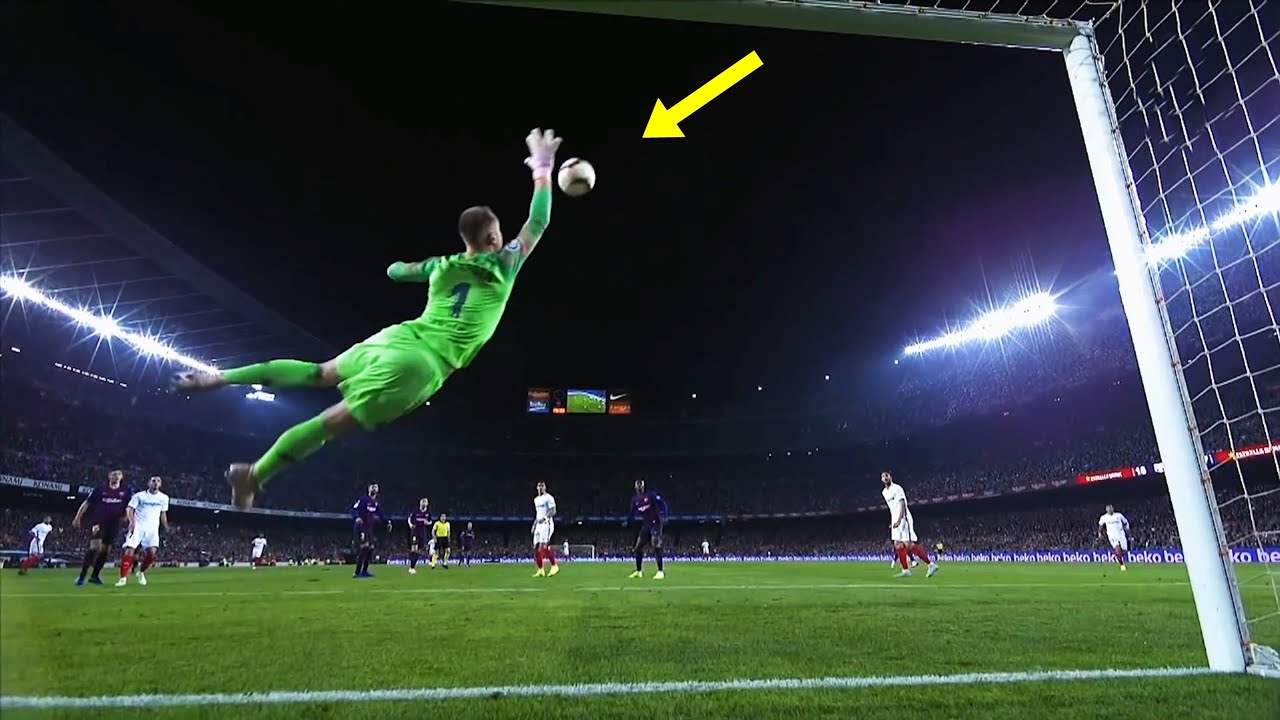The image captures a nighttime soccer game on a green grass field, with fluorescent lights illuminating the stadium. The scene is viewed from behind the goalie, who is mid-dive in a bright green jersey with the number one on the back, green shorts, green socks, and a white glove on his right hand. The goalie, with short dark hair, is airborne, reaching with his right hand to swat away a white soccer ball marked by a yellow arrow. The field is lined, indicating various areas of play, and players are visible wearing white jerseys with red socks, navy blue jerseys, and one player is in yellow in the background. Surrounding the field are stands filled with spectators under the night sky, with a scoreboard featuring the Nike logo visible in the distance. The edge of the white-framed goalie net is also discernible in the foreground.